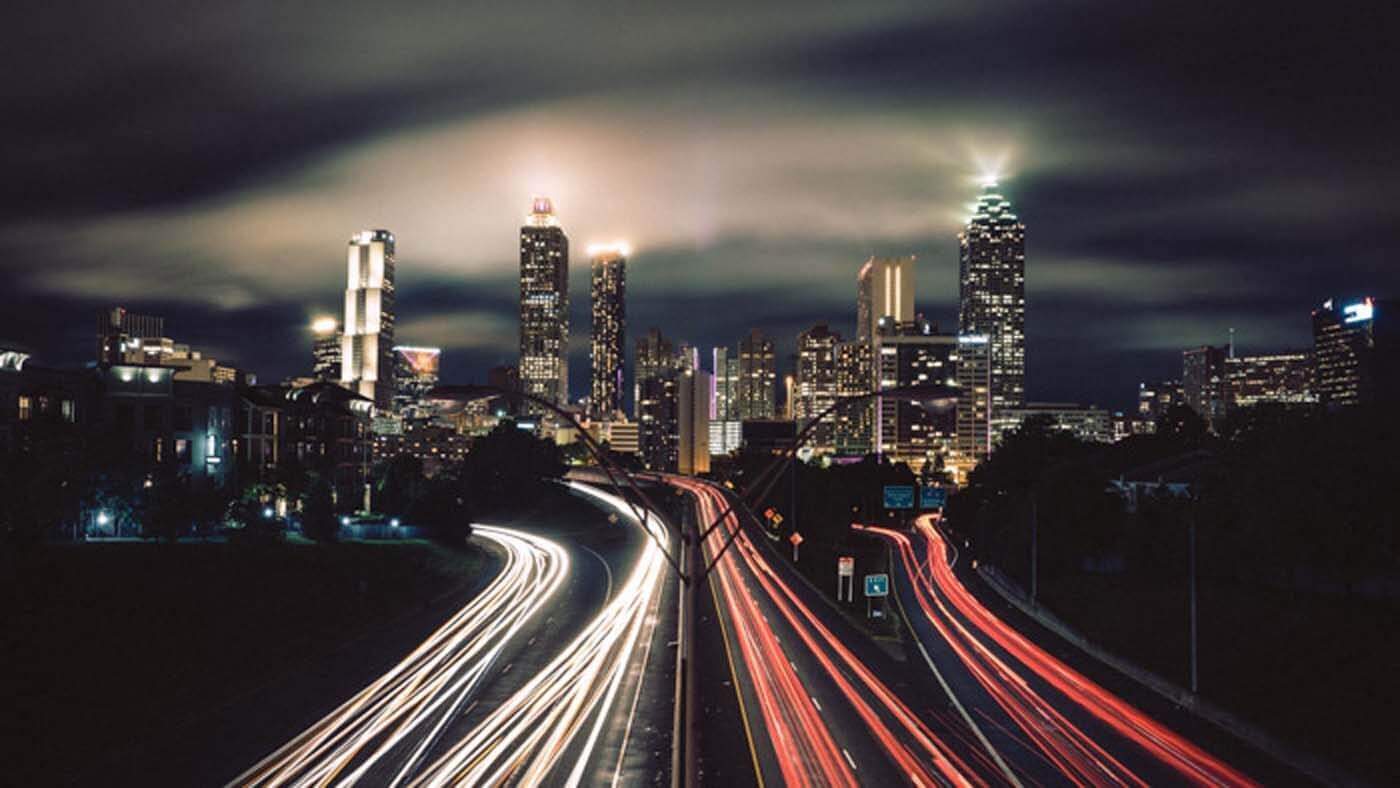This nighttime photograph captures a vibrant cityscape illuminated by shimmering skyscrapers and a network of light-trails created by a time-lapse exposure of traffic. The dark, somewhat cloudy night sky enhances the glow of the buildings, which appear to shine beams of light into the heavens. The image prominently features a complex highway system with visible signage and off-ramps, leading into the downtown area. Long neon ribbons of light—white from headlights and red from taillights—trace the curves of the roads, vividly depicting the flow of traffic moving toward and away from the city. The skyline is dominated by approximately 20 or so skyscrapers of various heights, each aglow with the bustling life within, further adding to the dynamic and vibrant character of the urban night scene.